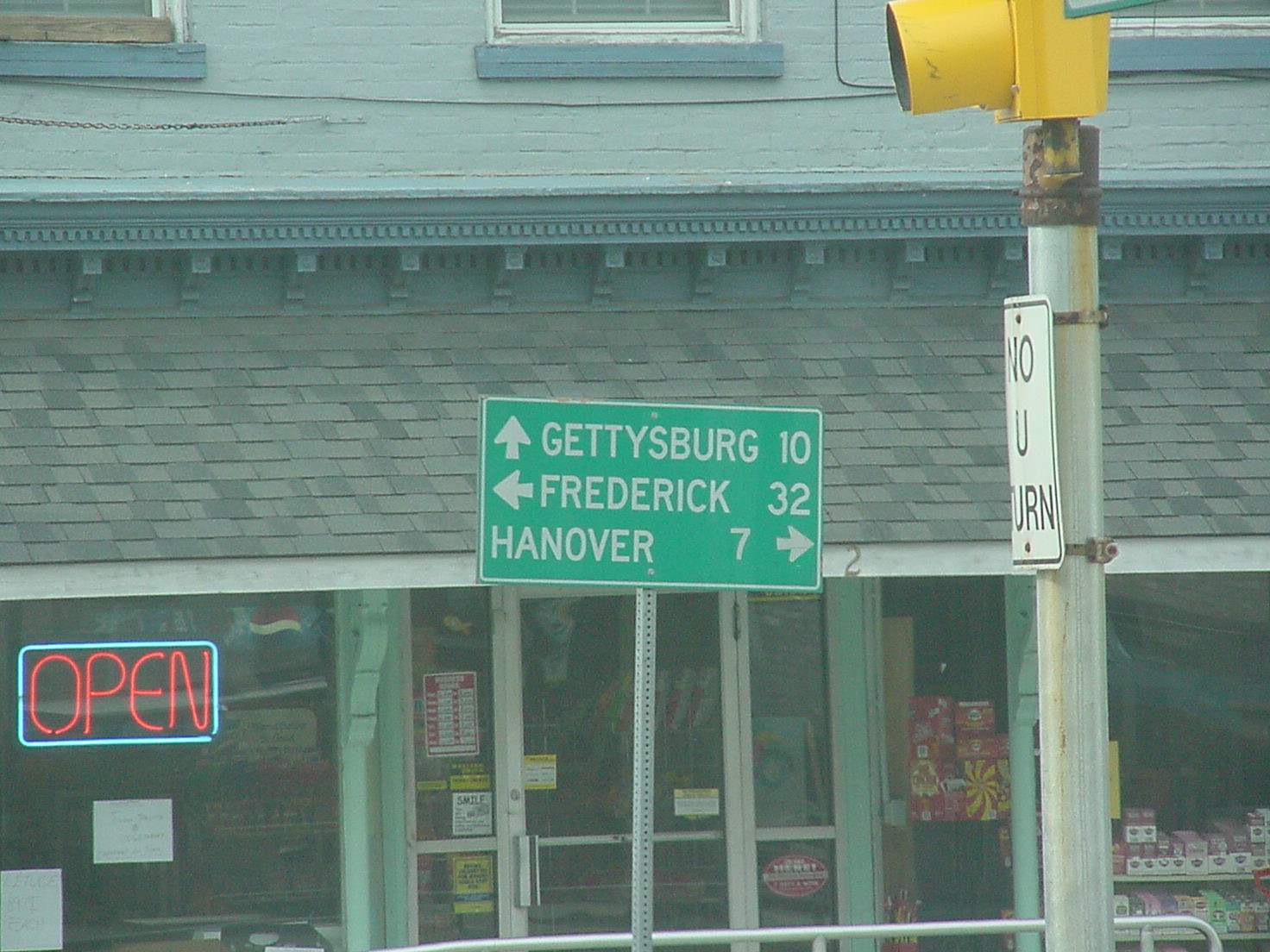The photograph captures a large building, likely a business, viewed from outside. Central to the image is a green street sign on a hollowed-out L-shaped silver pole. The sign lists distances to nearby locations with arrows: "Gettysburg 10↑", "Frederick 32←", and "Hanover 7→". The building features a glass door flanked by two glass windows, each supported horizontally by silver beams. Above these, the roof has alternating dark gray, mid-gray, and light gray shingles, with three visible window bottoms just beneath it. A neon "Open" sign with red lettering and a blue border sits against the left glass window. On the right, there's another large window showing red and purple boxes inside the building. Near the right side of the image, a metal pole with rusted areas supports a streetlight and a sideways white "No U-Turn" sign. The entrance includes a red rectangle sign with white rectangles likely indicating hours of operation, though the text is unreadable. The overall scene suggests a typical storefront with essential road signage and business identifiers.